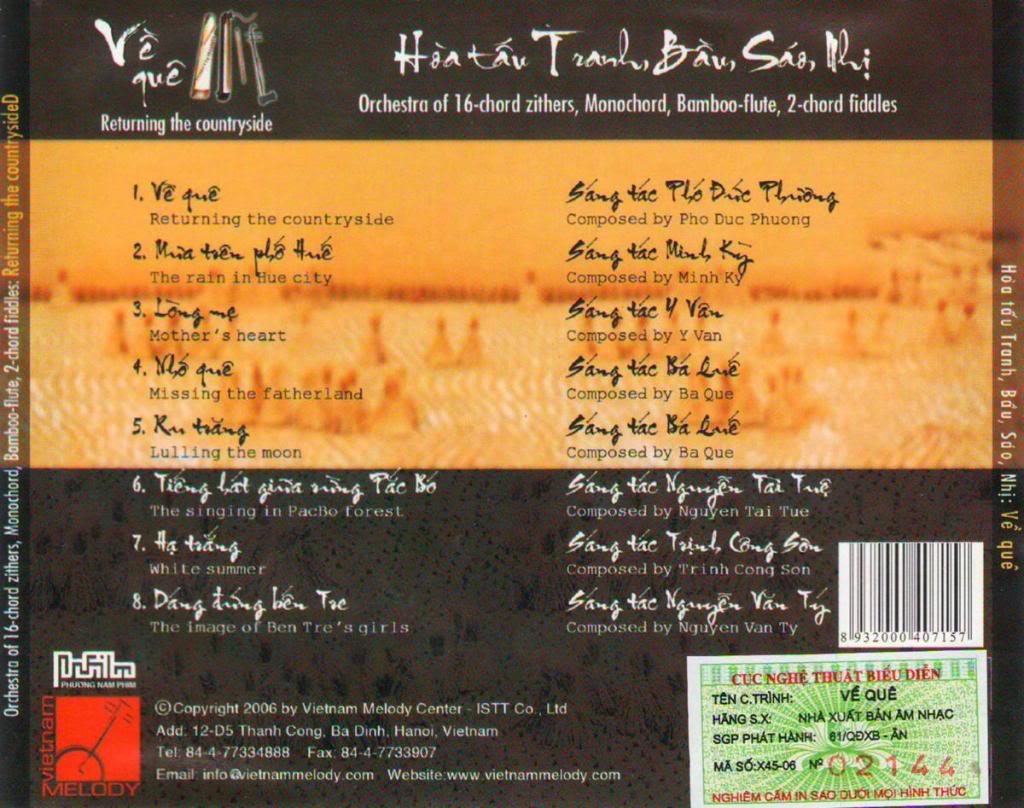This rectangular image, wider than it is tall, appears to be the program or back cover of a musical event or CD. The design is divided horizontally into three sections: a top brown area, a middle orange section, and a bottom brown background. At the top, in white lettering over a brown background, it lists the ensemble comprising a 16-chord zither, monochord, bamboo flute, and two-chord fiddles, with the title "Returning the Countryside" prominently displayed. The middle section features an orange background with a list of songs numbered one through five on the left and their composers on the right. The songs are: 1) "Returning the Countryside" by Phó Đức Phương, 2) "The Rain in Hue City" by Minh Kỳ, 3) "Mother's Heart" by Y Vân, 4) "Missing the Fatherland" by Bắc Kỳ, and 5) "Lulling the Moon" also by Bắc Kỳ. 

The bottom section, which has a brown background, continues numbering the tracks from six to eight with their respective composers: 6) "The Singing in Pak Bó Forest" by Nguyễn Thái Tử, 7) "White Summer" by Trịnh Công Sơn, and 8) "The Image of Bến Tre's Girls" by Nguyễn Văn Thái. The lower left-hand corner bears a red square logo with "Vietnam Melody" inscribed, and detailed contact information for Vietnam Melody Center, including their address in Hanoi, Vietnam, and various contact details such as phone, fax, email, and website. The lower right-hand corner features a white barcode directly above which lies a green ticket-like image containing black and red text, obscured by its non-English characters, recognizable by the numbers 0, 2, 1, 4, 4 in red. The primary language used in the text, aside from English translations of song titles, appears to be Vietnamese.